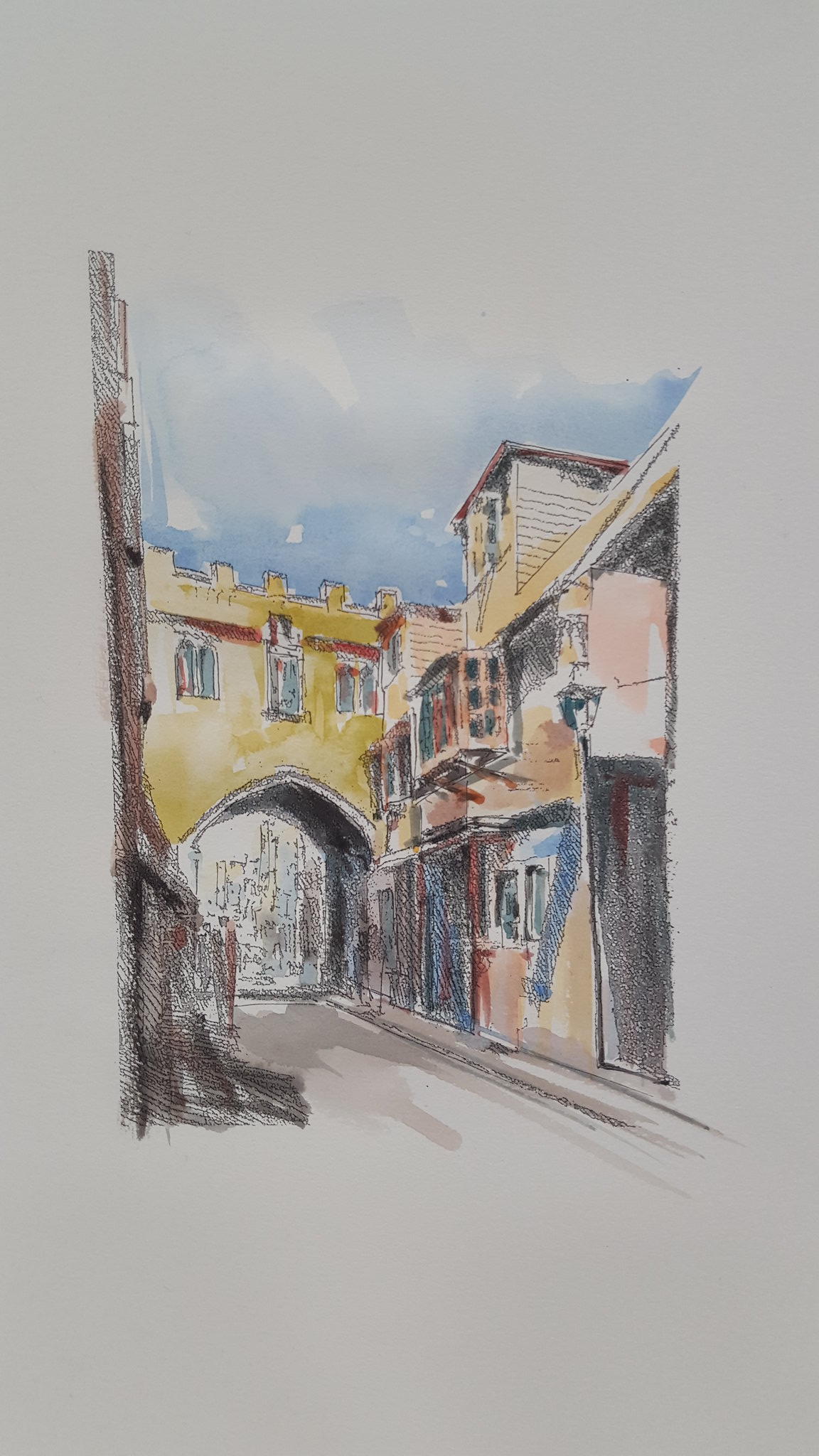The image depicts a detailed sketch on white canvas paper of a vibrant urban scene, reminiscent of an Italian street. Dominating the center is a yellow building with red accents, featuring three windows and a distinctive mini tunnel or archway at street level. This archway, painted gold, has a castle-like top and leads to a more minimalist representation of buildings in yellow and green hues, which lack specific details beyond their shapes. On the right side of the scene, there's a sequence of buildings in yellow, beige, and red tones, with some windows open and framed in white. A standout element on this side is a building with a projecting square-shaped window and a small upper level topped with a red triangular roof. On the left side, there is a partial view of a red and black building. The sky above is depicted in shades of blue with white clouds, and a brown and white road runs through the scene, intersecting under the archway.